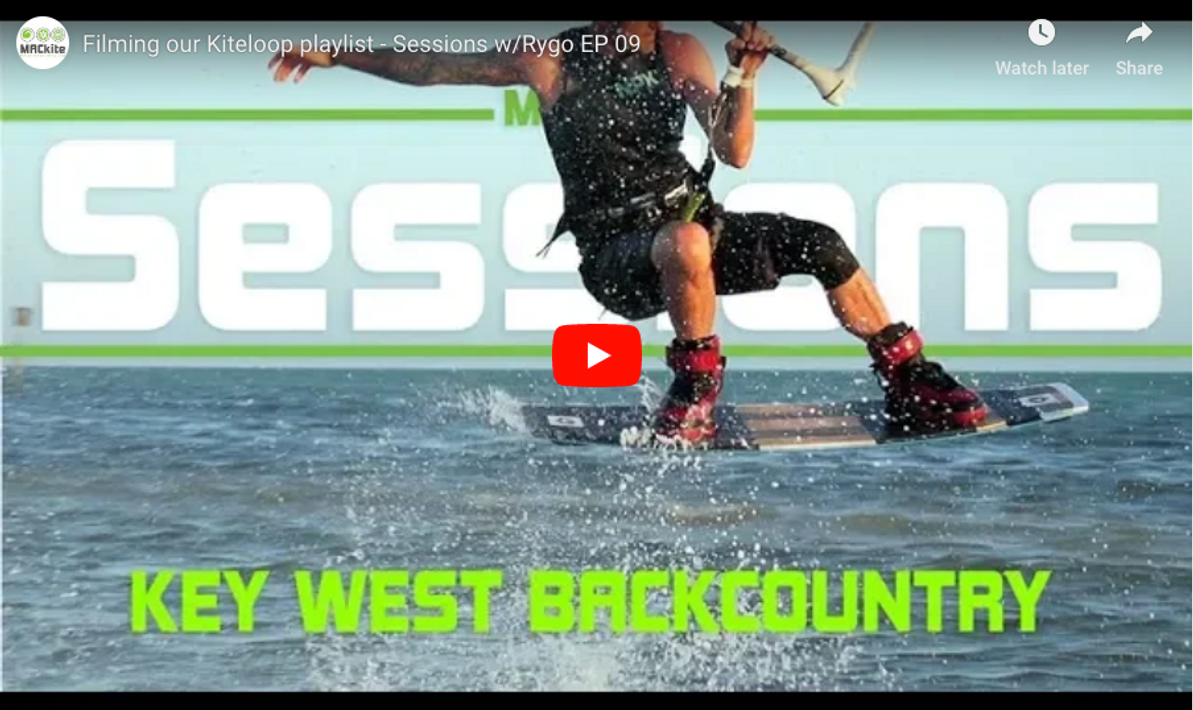The image is a screenshot from a YouTube video, titled "Filming our Kite Loop Playlist Sessions with Rigo EP09." It features a muscular man water skiing in the open ocean. The man is crouching on a water ski board, with his feet securely fastened in ski bindings. He is wearing black shorts and a black tank top. With his left hand, he firmly grips a tow rope attached to a bar that extends out of the frame. The text "Key West Backcountry" is prominently displayed in lime green letters at the bottom of the image. Behind the skier, on a light blue background, are white letters spelling "S-E-S-S" followed by the obscured letters behind the skier and "N-N-S." Icons for "Watch Later" and "Share" from YouTube are visible, as well as a red play button with a white arrow in the center of the image. The surface of the ocean is flat, glistening in shades of blue, with the man poised carefully to maintain his balance.